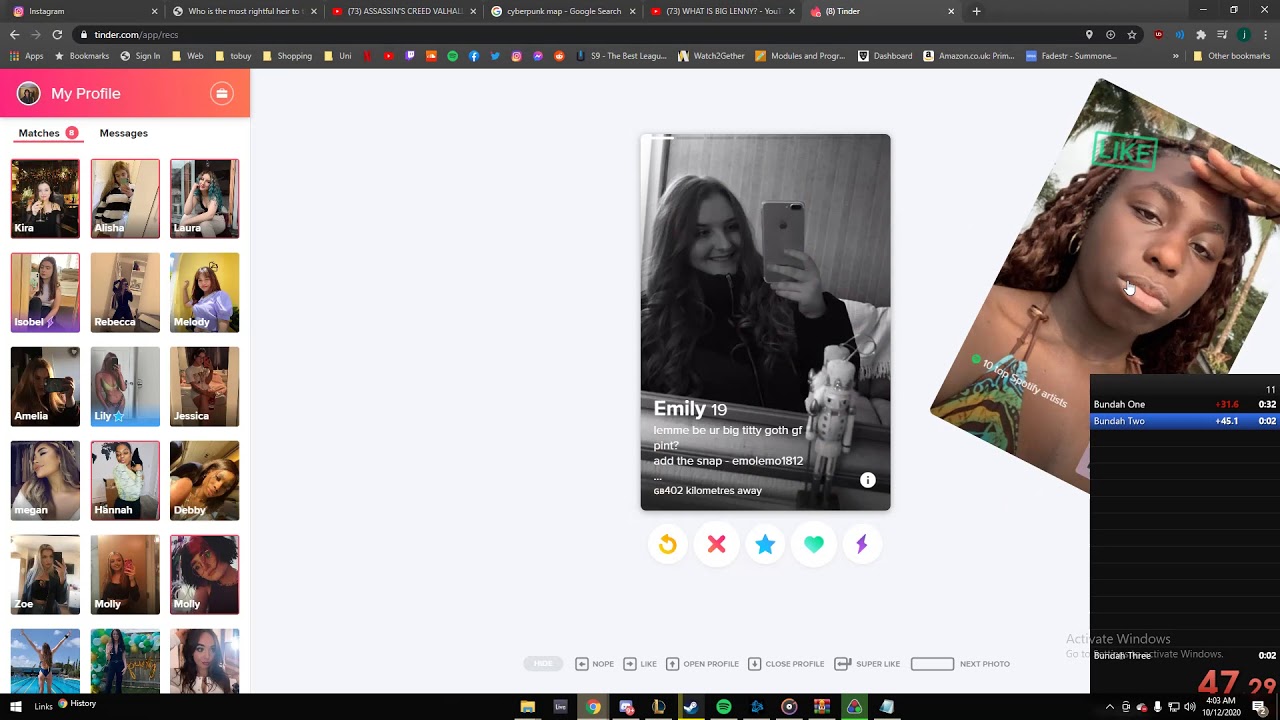**Caption:**

This screenshot depicts an open Safari web browser with multiple tabs. The active tab shows the Tinder web page, characterized by a peach-red background. At the top is the user's profile with an avatar on the left and a suitcase icon on the right. Under the profile heading, there are two sections: "Matches" with a pink underlined label and a pink circle indicating the number 8, and "Messages." Below "Matches," there are thumbnails of women's photos, three per row, totaling 18, showcasing a diverse mix of ethnicities, all appearing to be under 30.

On the right side pane, there's a black-and-white photograph of a 19-year-old named Emily. Her introduction reads, "Let me be your big, titty, goth, GF pint," along with her Snapchat screen name, EmoLimo1812. She is located 402 kilometers away from Great Britain and is pictured in a selfie wearing a turtleneck jacket in what appears to be a hotel room. Adjacent to her photo is a slanted image of a Black woman with a green 'like' stamp near her forehead, and below it is another pane listing users Buddha1 and Buddha2, followed by several numbers.

In addition to Tinder, the web browser includes the following tabs: Instagram, a search page titled "Who is the Most Rightful Heir To," a YouTube video of "Assassin's Creed Valhalla," a "Cyberpunk Map," and another YouTube video titled "What is Big Lanny."